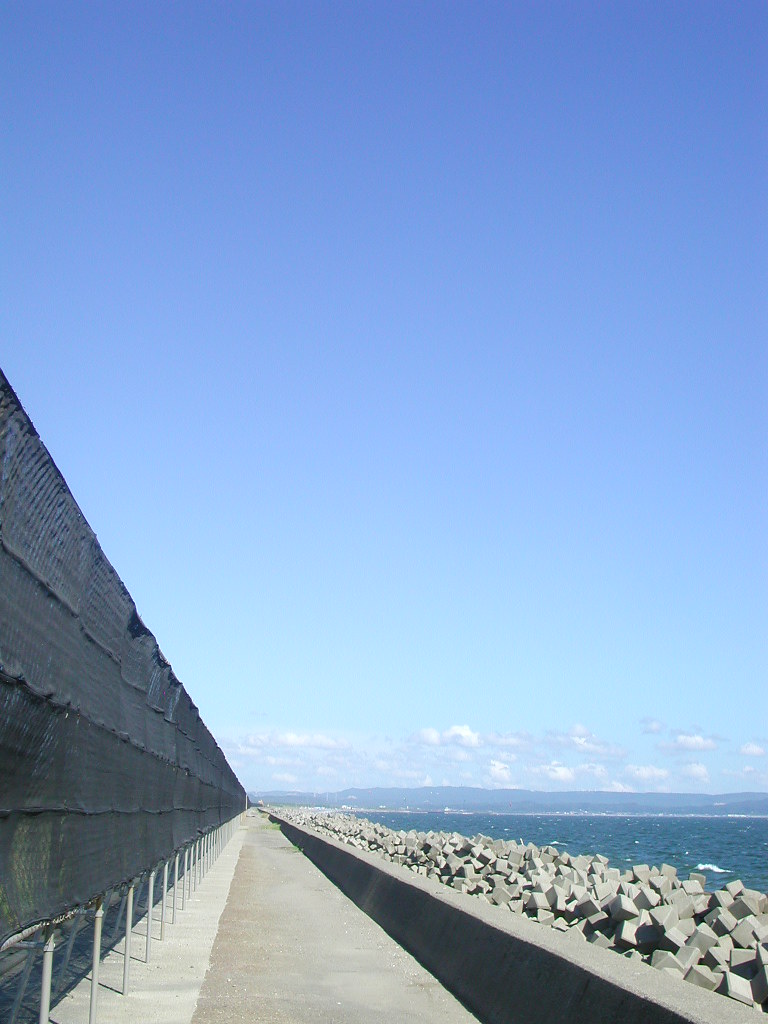The photograph, taken during the daytime, captures a picturesque scene of a seawall extending alongside a large body of blue water. Occupying the top half of the image is a clear blue sky, gradually transitioning to a deeper shade towards the top, with fluffy white clouds scattered along the far horizon. Hugging these clouds are distant, indistinct mountain ranges that add depth to the background. In the lower right corner, the blue water splashes against uniquely shaped, man-made blocks that create a breakwater. The center of the image features a long walkway running parallel to the seawall, bordered on the left by a tall black fence, comprised of stitched-together plastic and supported by gray metal rebar sticking up from the ground. This fence runs along the entire left side of the walkway, providing a boundary to the scene. The shadows cast by the seawall and fence create a contrast, emphasizing the bright, sunlit day depicted in the photograph.